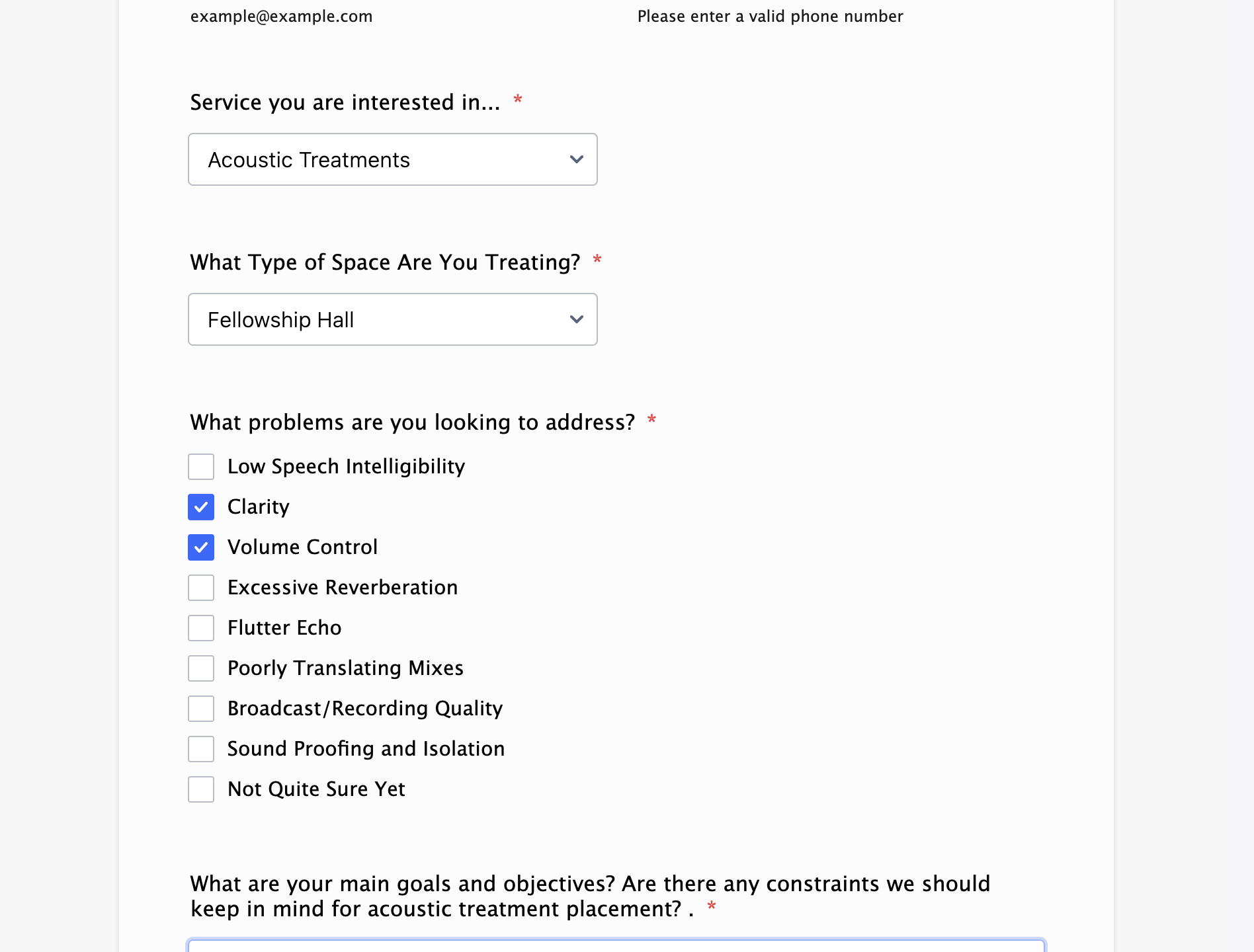The image features a user interface with a gray background and a prominent white pop-up box. The pop-up box is a form prompting the user for various details. At the top, it requests an email address with the placeholder text "example@example.com" followed by a reminder to "please enter a valid phone number." Below that, there is a drop-down menu labeled "Service you're interested in," which is currently set to "Acoustic Treatments."

Next, another drop-down menu asks, "What type of space are you treating?" with its current selection being "Fellowship Hall."

Further down, a section inquires, "What problems are you looking to address?" This section lists multiple issues with checkboxes beside each: low speech intelligibility, clarity, volume control, excessive reverberation, flutter echo, poorly translating mixes, broadcast/recording quality, soundproofing/isolation, and not quite sure yet. The options for "clarity" and "volume control" are the only ones selected, indicated by blue checkboxes with white check marks.

The final prompt asks, "What are your main goals and objectives? Are there any constraints we should keep in mind for acoustic treatment placement?" This text is intended for the user to provide further details relevant to their acoustic treatment needs.